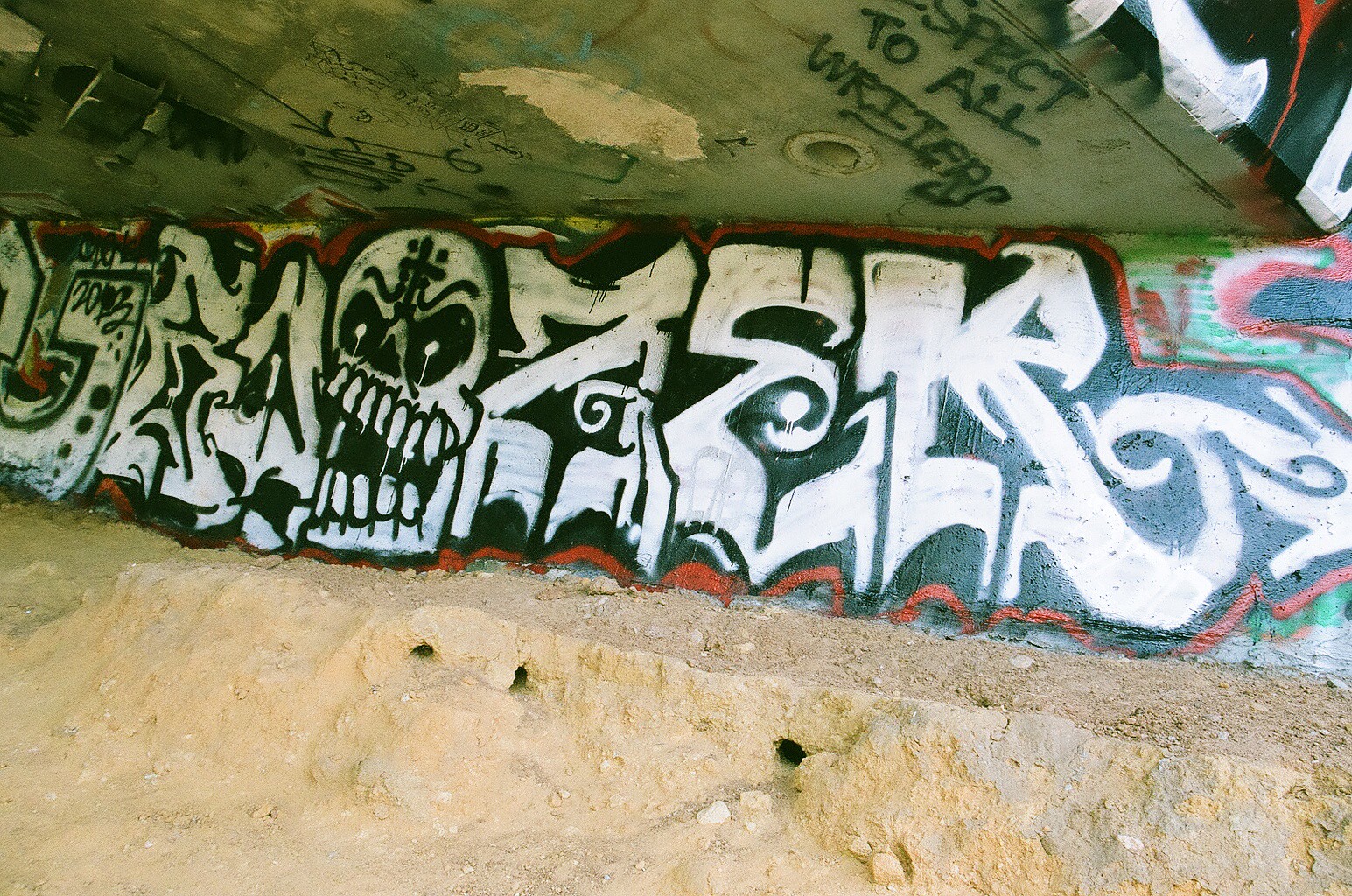The image depicts a detailed piece of graffiti on a concrete wall, likely situated beneath a highway bridge. The graffiti features the phrase "Respect to All Writers" in black paint, prominently displayed above the main artwork. The central section is a horizontal strip of stylized white letters outlined in black, with an additional red outline. Interspersed amongst the letters, a large skull with dark eyes and teeth occupies the center. The letters, which are difficult to decipher but possibly form the sequence "U, M, skeleton, Z, E, K," stand out against a black background with blue and green accents. The wall itself appears to be part of a dry riverbed or ramp structure, enhancing the gritty urban feel of the scene.